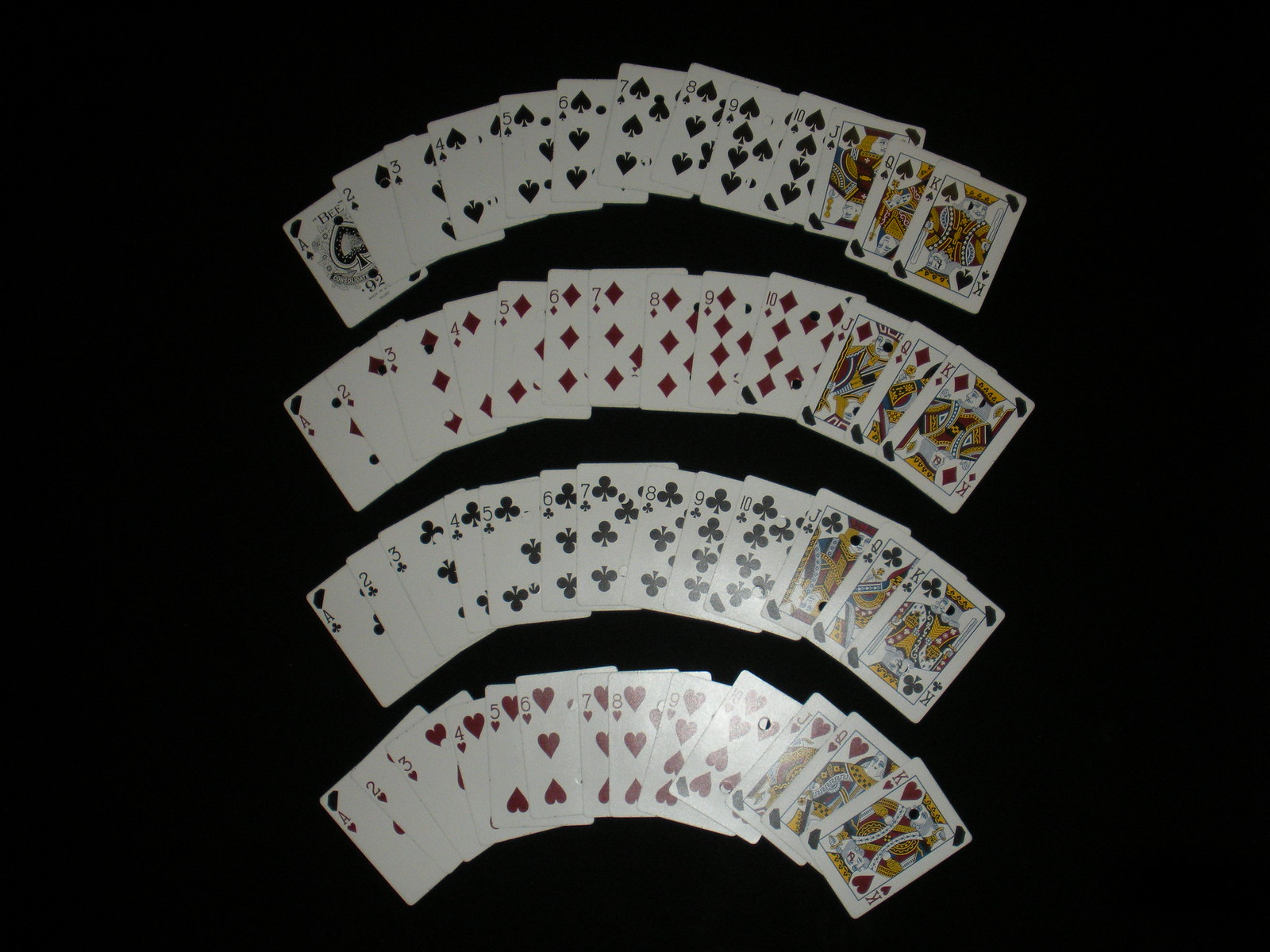A meticulously arranged photograph displays a full deck of playing cards against a dark, black surface. The deck is organized by suit, each spread out in a slightly overlapping pattern that creates a series of elegant, rainbow-like arcs. The suits are ordered from top to bottom as follows: spades, diamonds, clubs, and hearts. All cards, ranging from ace to king, are present and correctly ordered. Notably, the ace of spades features a more ornate design, possibly indicating the manufacturer of the deck. A soft glare from the camera's flash or the overhead light adds a subtle shine to the hearts suit, enhancing the visual interest of the scene. With no jokers in sight, the complete set of 52 cards is on full display.